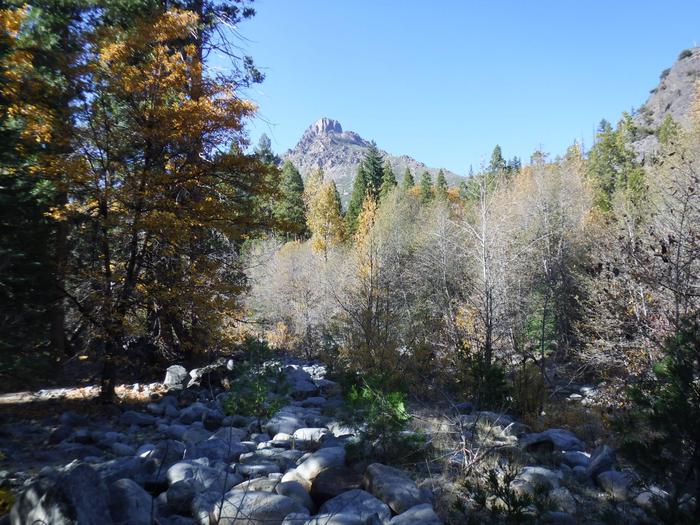This captivating photograph captures the serene beauty of a mountainscape in the early days of fall. Dominating the center background is a majestic, pyramid-shaped mountain with a rocky facade, framed by a crisp, cloudless blue sky. In the midground, a tapestry of trees showcases the seasonal transition: some are evergreen, some display leaves turning to a golden yellow, and others stand barren. In the foreground, a scattering of gray rocks suggests a dry riverbed, interspersed with weeds and plants. The array of colors—from the deep greens and yellows of the foliage to the browns and off-whites of the barren trees and rocks—emphasizes the depth and natural richness of this tranquil wilderness scene, perfectly captured in daylight.